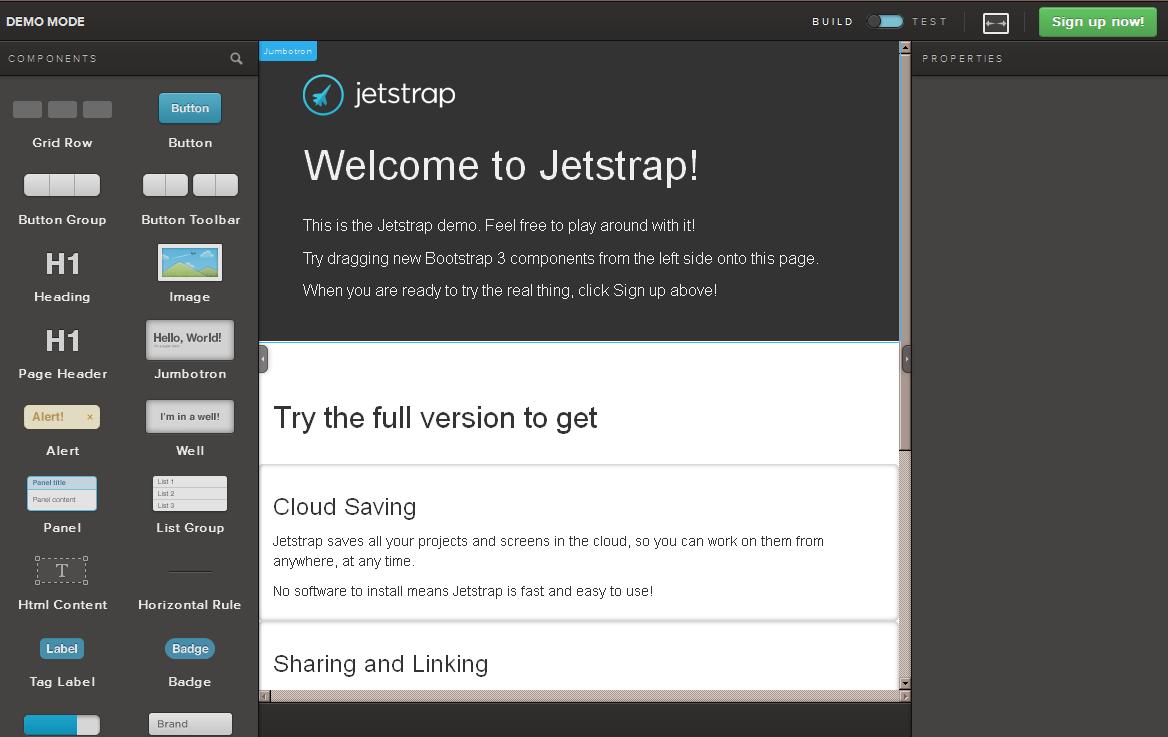**Welcome to the Chest Strap Demo Build**

Explore the unique features of Chest Strap with our interactive demo. Start by checking the green "Sign Up Now" button on the prominent jumbotron-style welcome screen. The demo interface is designed to let you freely experiment: drag and drop Bootstrap 3 components to see how they integrate into your projects.

When you are ready, try the full version to experience the full power of Chest Strap, including cloud saving, which allows you to save your projects and access them anywhere, anytime. The best part is there’s no software to install; simply click the provided link and start using it immediately.

Within the demo, you'll find various elements such as:

- **Grid Rows**: Organize your content seamlessly.
- **Blue Buttons**: Access different button functionalities including button groups and button toolbars.
- **Headings**: Add hierarchy to your content with H1 headings and page headers.
- **Images**: Incorporate visuals to enhance your project.
- **Alerts**: Utilize alert messages, like "I'm in a well panel," to capture user attention.
- **List Groups and HTML Content**: Create structured and versatile content blocks.
- **Horizontal Rules**: Separate sections for better readability.
- **Labels and Tags**: Implement label tags and badges for easy identification and categorization of elements.

Dive in and harness the potential of Chest Strap to make your project effortless and accessible.